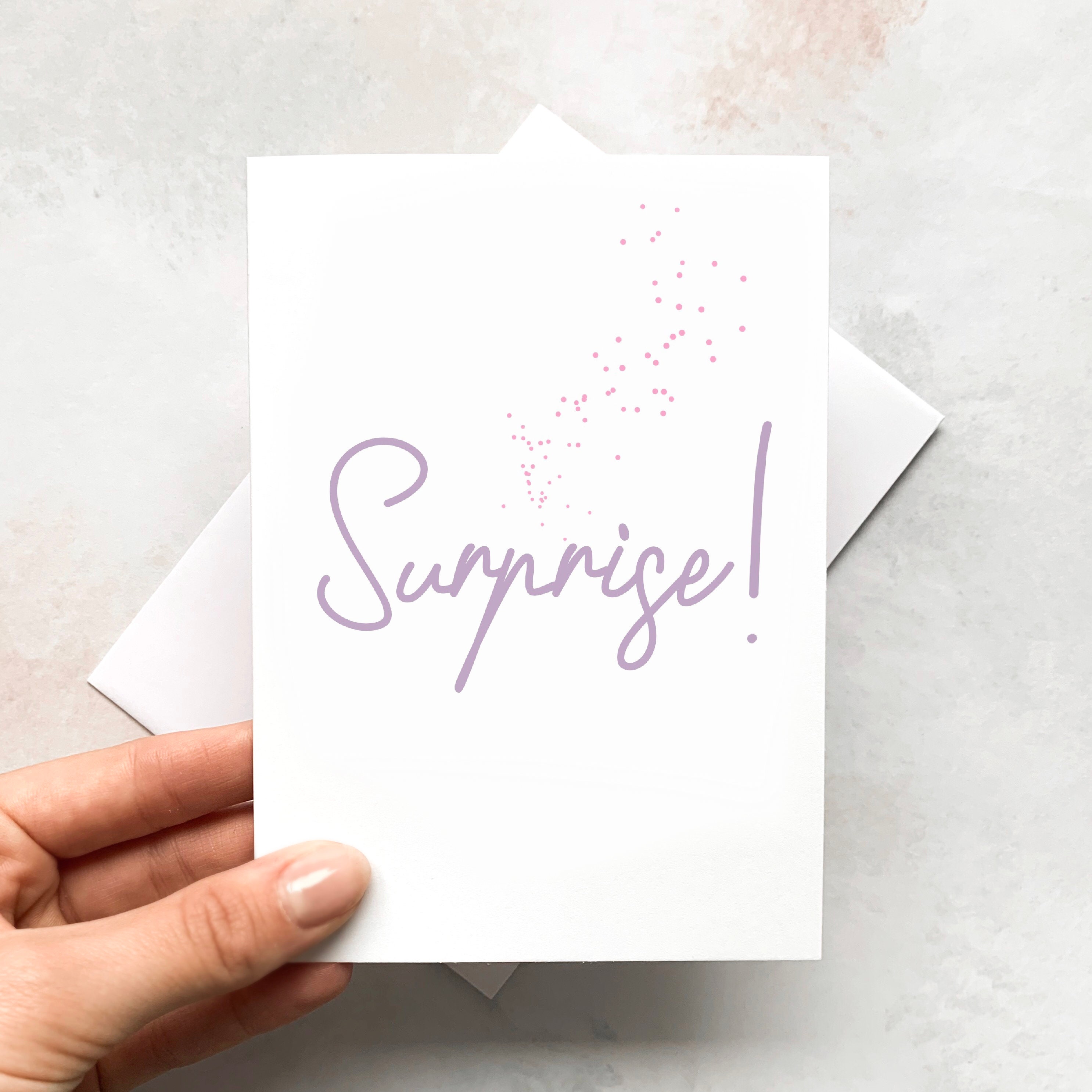In this photograph, a Caucasian woman's hand with naturally colored but glossy polished nails is holding a white greeting card. The card, displayed in a vertical rectangle, features the word "Surprise!" in light purple script at the center. Above the text, tiny light purple confetti dots cascade towards the top right corner. The hand holding the card is positioned at the bottom left of the image, with the thumb facing upward and fingers clasped behind the card. The background is predominantly white, with a slight gray tint and a beige powder-like texture near the top. A white envelope is partially visible behind the card, tilted at about a 30-degree angle. The entire scene rests on a subtle marble-like surface, adding to the clean, minimalist aesthetic typical of a stock photo.